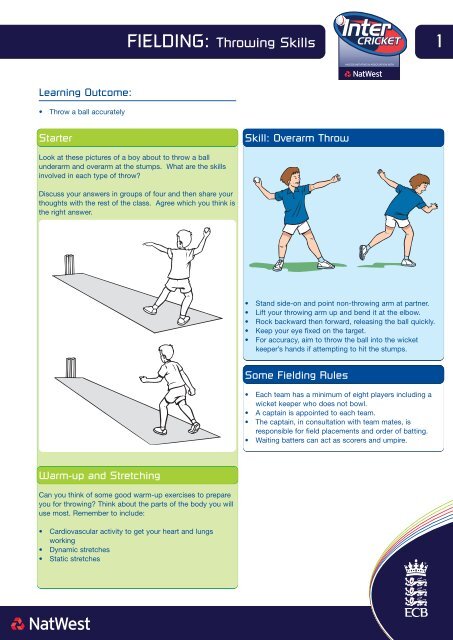This image is an informational sheet presented by NatWest and the ECB about fielding throwing skills in cricket, specifically designed for newcomers to the game. At the top, it reads "Fielding: Throwing Skills - Inter-Cricket" with a focus on learning outcomes aimed at teaching accurate ball control. It instructs on both underarm and overarm throws, illustrated with diagrams of a young boy in a blue short-sleeved shirt, white shorts, and white shoes demonstrating each type of throw.

The left side of the image shows sequences of the boy preparing to throw and completing the throw, while the right side provides detailed step-by-step instructions for the overarm throw: standing side-on, pointing the non-throwing arm at the target, lifting and bending the throwing arm at the elbow, rocking backward then forward to release the ball quickly, and keeping the eyes fixed on the target. It highlights accuracy and recommends aiming the ball into the wicket-keeper's hands to hit the stumps effectively.

The sheet also prompts group discussion among four participants to identify the skills involved in each type of throw and reach a consensus on the correct techniques. Warm-up exercises, including cardiovascular and stretching activities, are emphasized to prepare the body for throwing. Additionally, the document outlines basic fielding rules, including team composition and roles, such as the appointment of a captain responsible for field placements and batting orders.